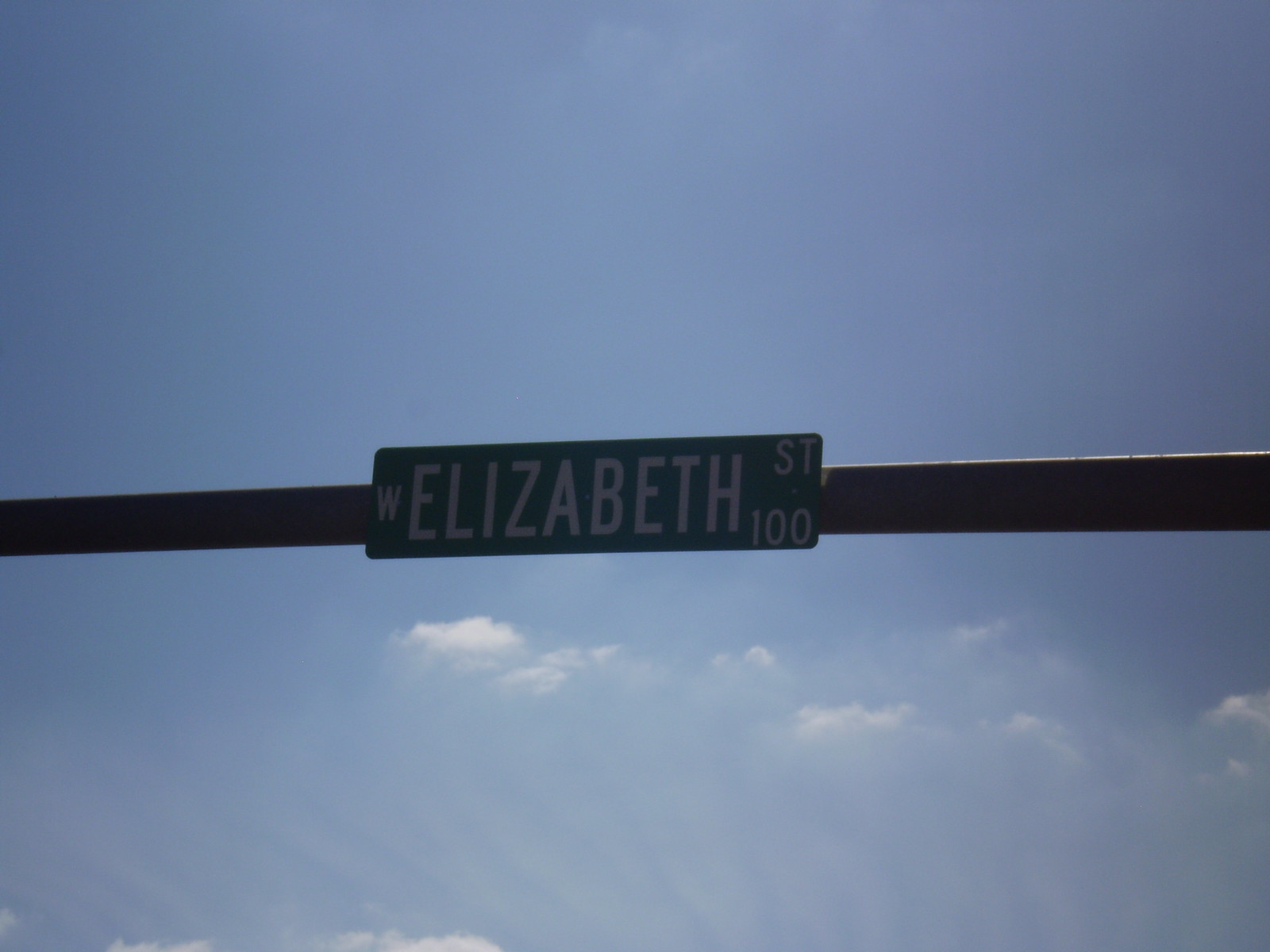This photograph captures an idyllic scene featuring a street sign against a pristine blue sky. The sky is flawlessly clear, save for a few wispy clouds drifting in the lower left-hand corner. Dominating the center of the image is a black street sign pole stretching horizontally across the frame. Attached to the pole is a green street sign trimmed with white, displaying the text "West Elizabeth Street 100." The sign is detailed with a diminutive "W" for West at the top, a bold "Elizabeth" in the middle, a small "Street" in the upper left corner, and a small "100" at the bottom left corner. The serene background and the precise composition of the street sign make this a visually appealing and tranquil image.